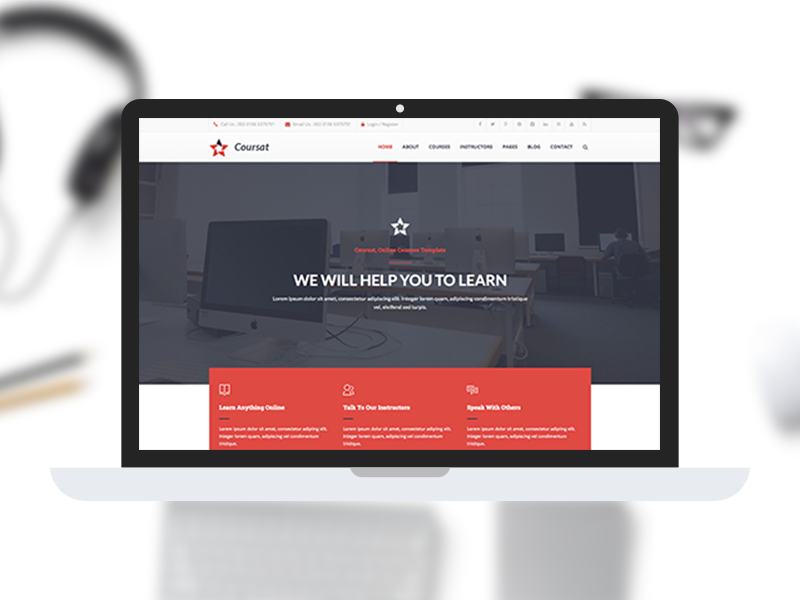This is a color image of a stylized, infographic-like representation of a laptop. The laptop’s screen, bordered by a black band, displays a web browser with various elements that are difficult to read due to the small size and blur of the image. The laptop's base is grey. The background is blurred, and various items are scattered around the laptop: on the left side, there is a pair of headphones, a black pen, and a yellow pen or pencil. On the lower right corner under the laptop, there is a pair of glasses and an indistinguishable grey object. The web browser open on the laptop shows multiple tabs at the top, accompanied by a logo on the left side featuring a star with one black point and the remaining points in red. To the right of the logo, the word "Corset" is written in black. On the right side of the browser window is a list of tabs with "Home" prominently marked in red. The central image within the browser appears to be a computer lab with several Mac computers, occupied by a person in the upper right corner facing away. Overlaying this image, in the middle, is a star logo and a line of white text stating, "We will help you to learn." Further down, there is an orange rectangle with unreadable white text and a white band at the bottom on both left and right sides.